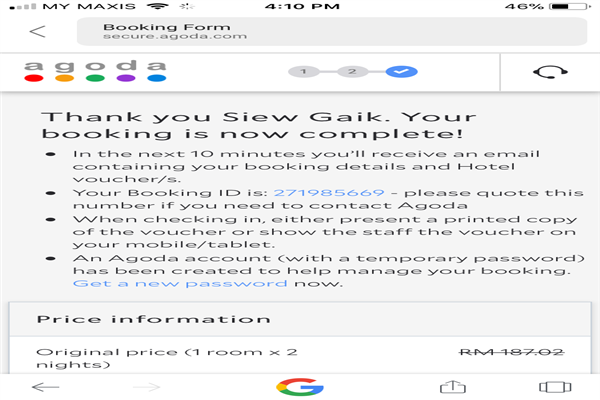The image showcases a webpage with a gray background at the top, featuring the text "My Maxis" on the left and the time "4:10 p.m." in black in the center. On the right, a battery icon indicates a 46% charge. Below this header, a gray bar displays the URL "booking forum secure.agoda.com."

The main section of the page features the "Agoda" logo, with each letter in a distinct circular color: red, yellow, green, purple, and blue. Below the logo, the numbers "1" and "2" are shown, followed by a blue circle containing a white checkmark, indicating a completed step.

The text beneath the checkmark reads: "Thank you, SIEW GAIK. Your booking is now complete." Further details explain that an email will be received within the next 10 minutes, containing booking information and hotel vouchers. Additional information follows regarding the booking ID and check-in instructions.

Further down, the price details section includes:
- Original price (1 room x 2 nights): RM 187.02 (crossed out).

At the bottom left, there is a thin gray arrow pointing to the left, and in the middle, the colorful Google "G" symbol is visible.